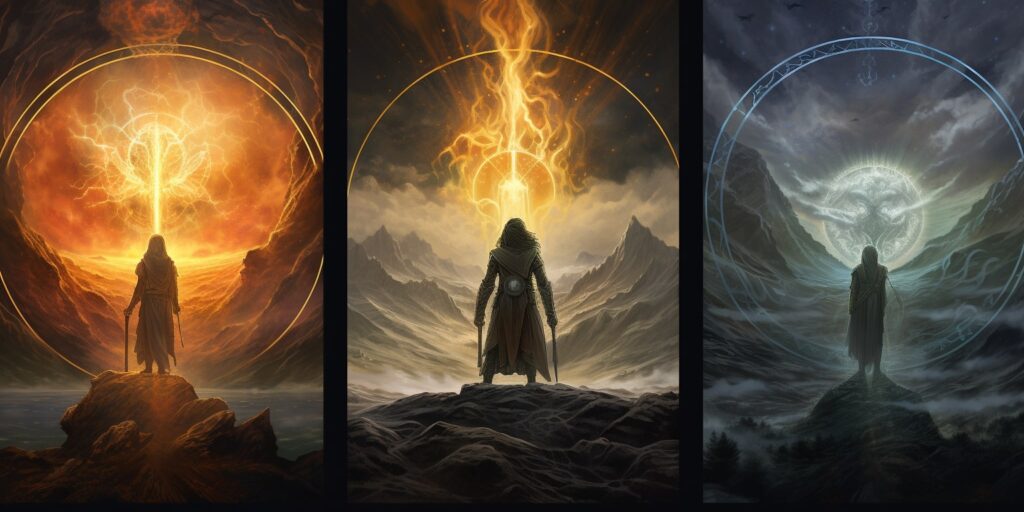The image is a computer-generated painting depicting a triptych, with each of the three frames showcasing a similar yet distinct scene. Each frame features a silhouetted figure standing on a rock, resembling the peak of a mountain. The first frame shows a robed figure holding a staff in their left hand and a sword or wand in their right. This figure faces an orange and yellow landscape filled with water and flanked by mountains. Fire shoots up and rains down from the sky, creating a dramatic scene where lightning forms a line with a circle around it, all enclosed by a yellow sphere.

In the middle frame, a person, possibly wearing a robe and gloves with a circular symbol on their back, wields two swords. Standing among gray rocks and similarly hued mountains, this figure faces a yellow-orange lightning shape that arcs around a half-circle in the sky, continuing the fiery motif.

The third frame diverges as its focal figure, no longer holding any weapon, stands amidst a blue-themed, fog-enveloped landscape with mountains in the background. Instead of fire, this scene features a serene moon encircled by white, with dark shapes that could be birds or bats adding to the mystical ambiance. Despite the absence of fire, the sense of standing before an alien mountain landscape unifies all three images.